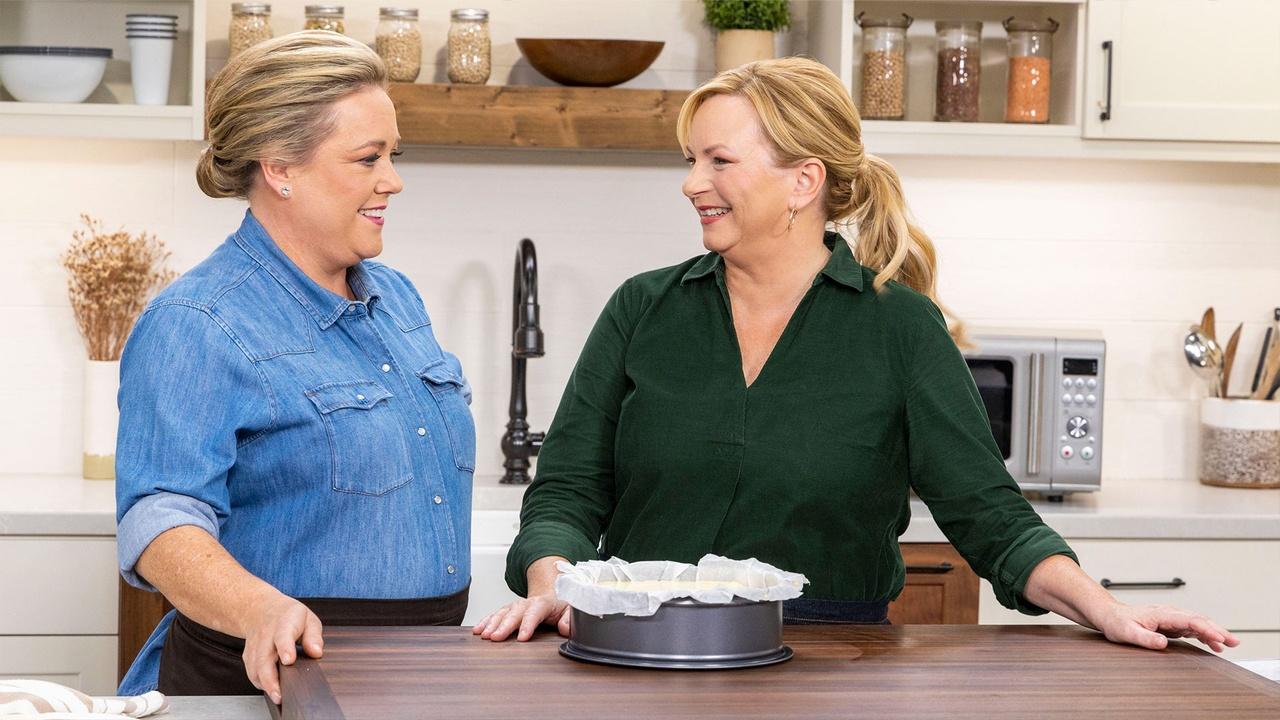This photograph depicts a scene from America's Test Kitchen featuring two blonde, somewhat overweight women chefs engaged in a friendly conversation while preparing something. The woman on the left is wearing a long-sleeve denim shirt with her sleeves rolled up and a black apron around her waist, looking towards the woman on the right. The woman on the right is dressed in a green, thick canvas shirt, also with sleeves rolled up, and appears to be wearing blue pants. Both women are smiling and enjoying the moment.

In front of them, on a thick, dark cherry or mahogany-stained butcher block countertop, sits a round, pewter cake tin lined with wax paper. The spacious, well-lit kitchen backdrop features a gray, metallic-looking pull-down faucet with a swan neck design, perfectly arched over the sink. To the right of the faucet is a silver stainless steel microwave. A vase with yellow, dried flowers, possibly wheat, sits to the left, adding a rustic touch.

Above the faucet, a wooden shelf showcases an array of items: several glass mason jars containing tan, black, and red ingredients; a succulent plant; a wooden bowl; and some spice jars in a three-tier wooden cubbyhole. To the left of the shelf, there's a set of white bowls and cups with black rims. The clean, white kitchen cabinets with black handles frame the scene, enhancing the overall aesthetic. The background also features a utensil pot containing both silver and wooden tools, adding to the kitchen's functionality and charm.